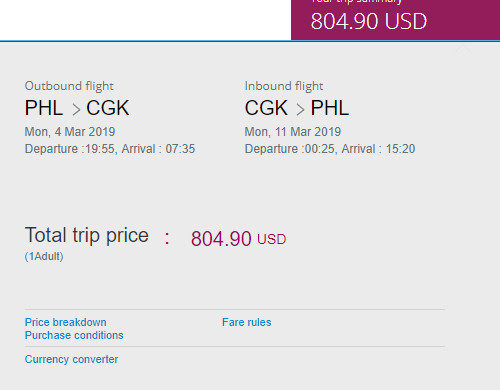The image features a gray background with a small purple box located at the top-right corner. Inside the purple box is a white text displaying "804.90 USD."

In the gray section, there is informative text without any visible borders, resembling a box layout. The first section is titled "Outbound Flight." Beneath this heading, bolded text states "PHL" followed by an arrow pointing to "CGK." Below these abbreviations, the text details the flight schedule: "Monday, March 4th, 2019," with departure at "1955" and arrival at "0735."

Opposite this text is another block of information with a similar format, titled "Inbound Flight." It reads "CGK" followed by an arrow pointing to "PHL." The return flight details are listed as "Monday, March 11th, 2019," with departure at "0025" and arrival at "1520."

Below these sections, slightly to the left, the text "Total Trip Price" is displayed, with a subnote in parentheses stating "(1 Adult)." Directly across from "Total Trip Price" in purple text is "804.90 USD."

Further down, there are two horizontal lines, between which blue text spells out "Price Breakdown, Purchase Conditions, Fare Rules." Below the second line, "Currency Converter" is also displayed in blue text.